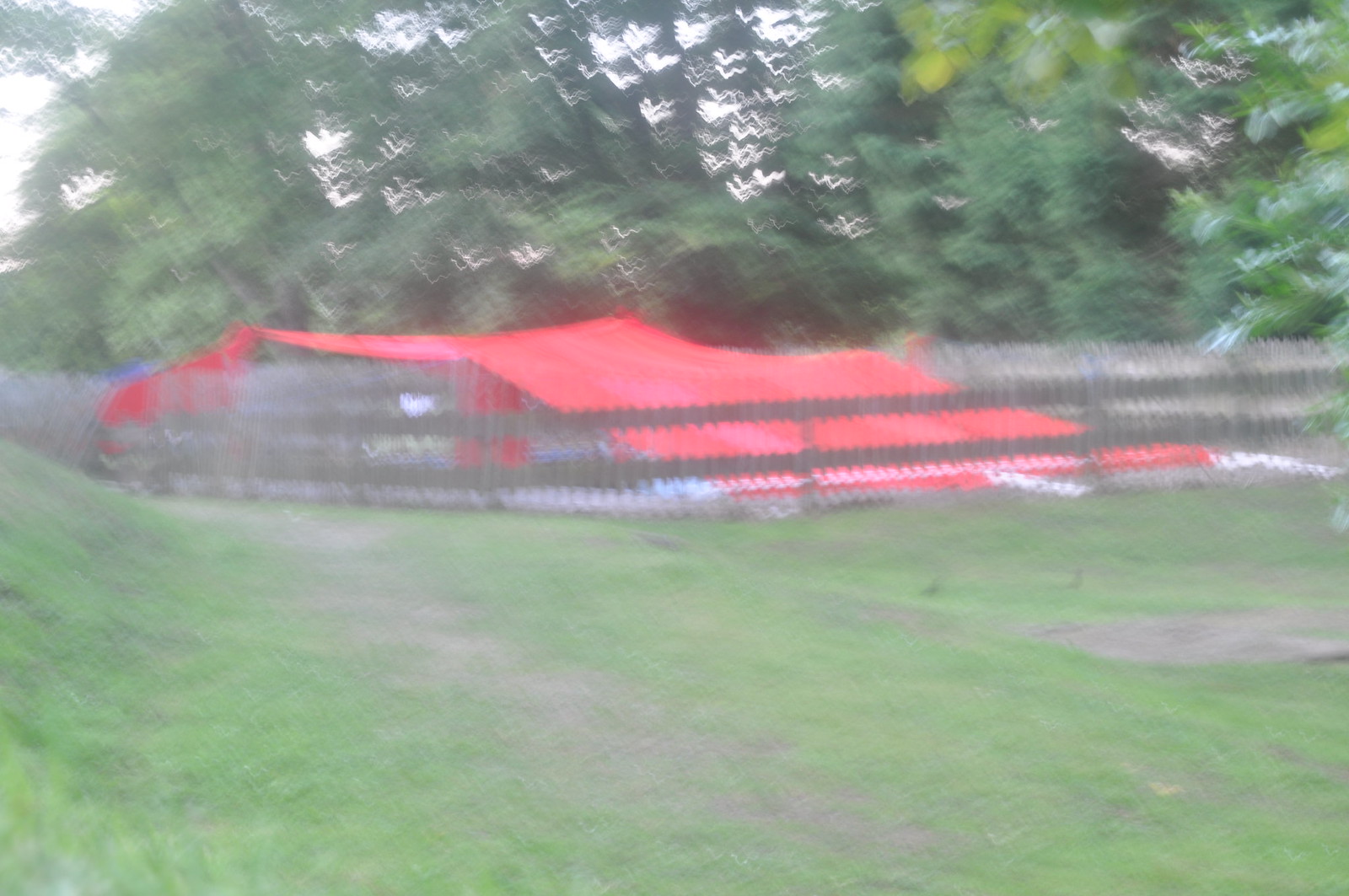This is a somewhat blurry, daytime outdoor photograph featuring a flat green grassy area interspersed with worn footpaths. Central to the image is a fenced-in structure, seemingly square in shape, with a reddish tarpaulin roof supported by poles covering what appears to be a shallow excavation or similar ground disturbance. The fence around this area consists of sturdy posts and double horizontal beams. In the background, a cluster of green trees meets a light, slightly overcast sky, creating a natural, serene backdrop. The overall scene suggests a possibly rural or farmland setting.